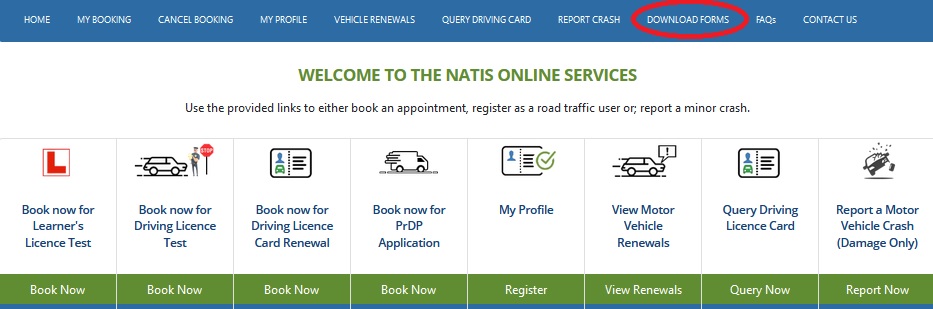The image is a narrow, horizontal section capturing the top portion of a website interface. At the very top, there is a slim, horizontal blue banner featuring various navigation options in white text: "Home," "My Booking," "Cancel Booking," "My Profile," "Vehicle Renewals," "Query Driving Record," "Report Crash," "Download Forums," "Fax," and "Contact Us." Notably, the "Download Forums" option is emphasized with a red circle around it.

Just below this banner, centered on a white background, is a welcoming message in green, all-uppercase text: "WELCOME TO THE NATIS ONLINE SERVICES." Directly beneath the welcome message, instructions are given in a smaller font, urging users to "Use the provided links to either book an appointment, register as a road traffic user, or report a minor crash."

Further down, the webpage is divided into eight distinct, rectangular blocks arranged side by side. Each block contains a different service option in bold letters:
1. "Book Now for Learner's License Test"
2. "Book Now for Driver's License Test"
3. "Book Now for Driving License Card Renewal"
4. "Book Now for PRDP Application"
5. "My Profile"
6. "View Motor Vehicle Renewals"
7. "Query Driving License Card"
8. "Report a Motor Vehicle Crash, Damage Only"

The layout appears streamlined to facilitate user navigation and access to various online services offered by NATIS.